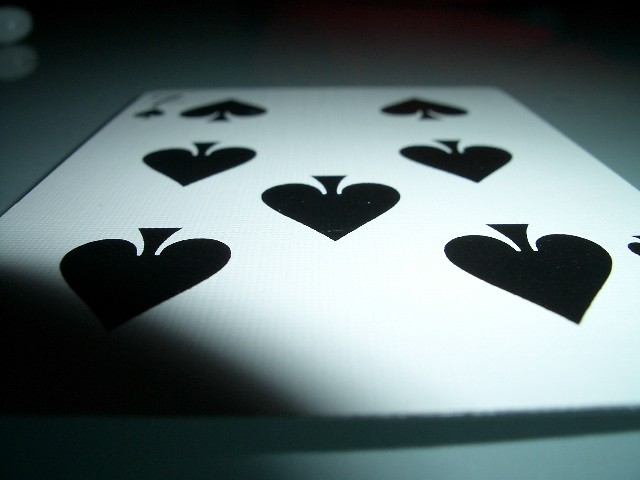The image features the Seven of Spades playing card lying relatively flat on a grayish background with a slight hint of green. The upper left-hand corner of the card displays the number "7" and spade symbol. The card is heavily shadowed in the lower left or "southwestern" corner, with lighter shadowing elsewhere, obscuring parts of the card slightly. The spade symbols are upside down, with their points facing the viewer. Interestingly, the seventh spade is positioned closer to the viewer rather than being centrally located among the three spades on either side. The overall scene is simple, with the dark background contrasted by the card's grayish foreground.